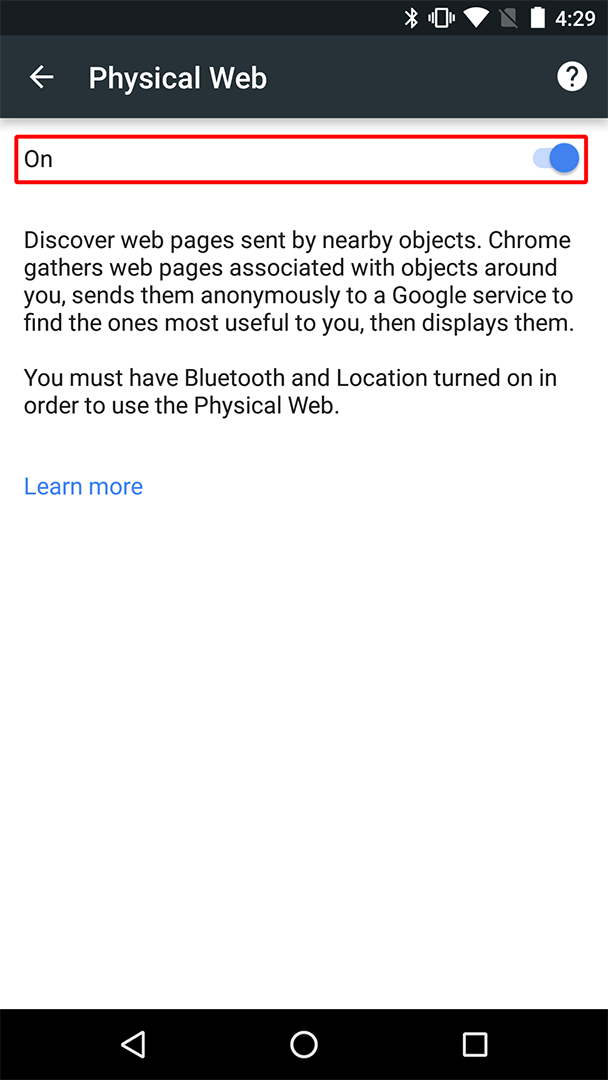This is a detailed screenshot of the settings section within a specific app on a mobile phone. 

**Top Status Bar:**
- On the top right-hand corner, a series of status icons are displayed, including Bluetooth, an iPod icon, a possible screen extension icon, Wi-Fi, battery level, and the current time (4:29).

**Title Section:**
- Just below the status bar, the app's title "Physical Web" is shown in white font. 
- To the left of the title, there is a back arrow for navigating to the previous screen.
- To the right of the title, a question mark icon provides help or additional information.

**Settings Toggle:**
- Following the title section, there is a settings option labeled "On" with a toggle switch positioned to the far right, which can be turned on or off. This section is outlined in red.

**Informational Text:**
- Below the toggle switch, the app explains in black font: 
  "Discover web pages sent by nearby objects. Chrome gathers web pages associated with objects around you and sends them anonymously to a Google service to find the ones most useful to you, then displays them. You must have Bluetooth and location turned on in order to use this Physical Web."
- At the end of this explanation, "Learn more" is highlighted in blue, indicating a link to additional information.

**Navigation Bar:**
- At the bottom of the screenshot, the phone's navigation buttons are visible: a back arrow (triangle pointing left), a circle (home), and a square (recent apps).

This detailed imagery captures the entirety of the mobile interface, focusing on the settings for the Physical Web feature within a specific app.